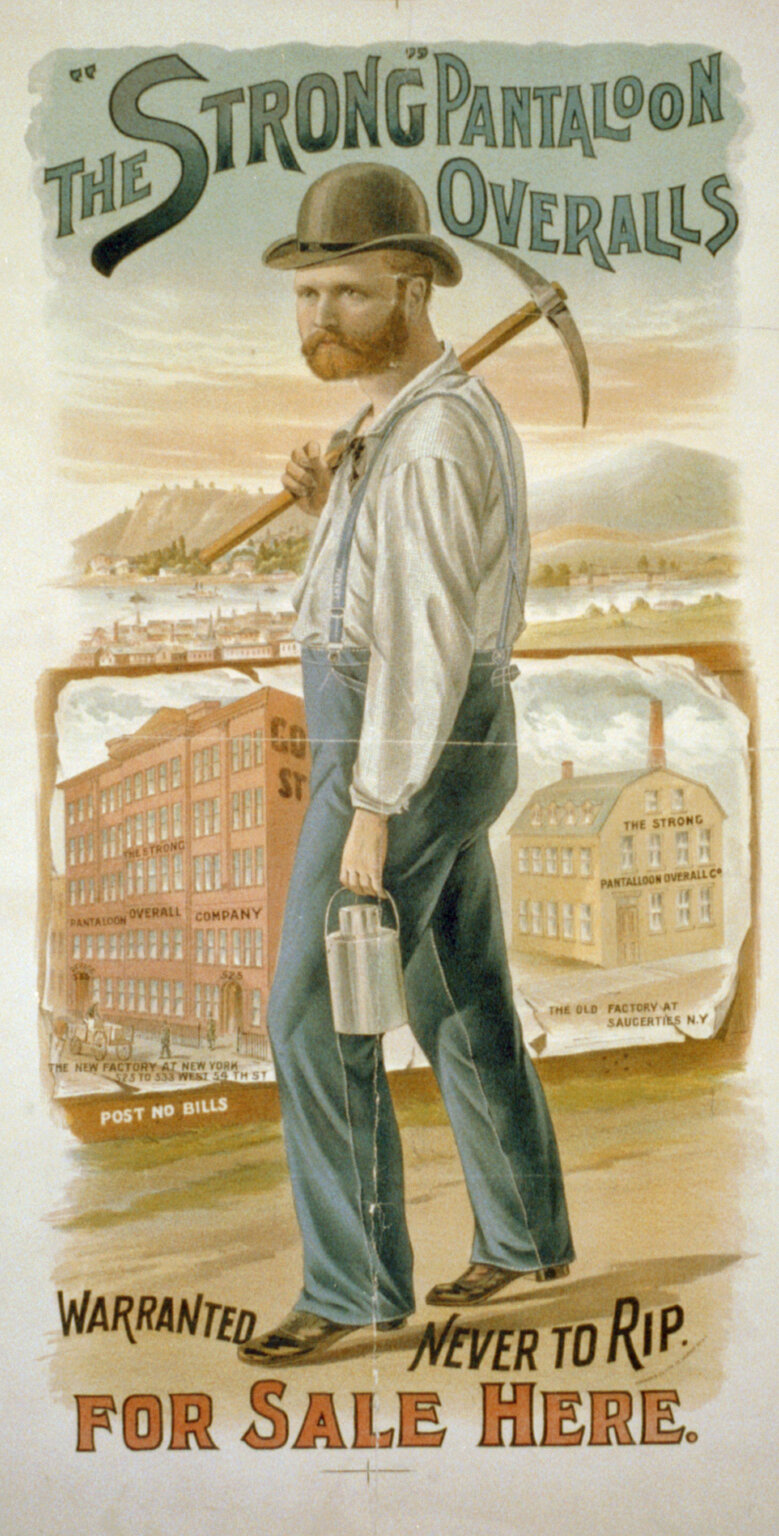This vintage advertisement poster, likely from the early 20th century, features a vividly colored illustration of a rugged, bearded man with a reddish mustache. He stands at the center wearing a derby hat, blue overalls, a white shirt, and black boots. He holds a pickaxe over his right shoulder and a flask in his left hand, embodying a "salt-of-the-earth" character. Above him, the poster reads in prominent blue text, "The Strong Pantaloon Overalls," and below him, in black and red text, it proudly announces, "Warranted Never to Rip. For Sale Here."

In the background, there are two large buildings—a five or six-story factory labeled "The Strong Pantaloon Overall Company," and another three-story building resembling a barn. Both buildings suggest a manufacturing setting, with additional details like a "Post No Bills" sign enhancing the nostalgic feel. The overall scene is set against a beautifully painted backdrop depicting mountains, a bay, and possibly row houses, done in soft greens, grays, and reds, giving depth and context to the advertisement.